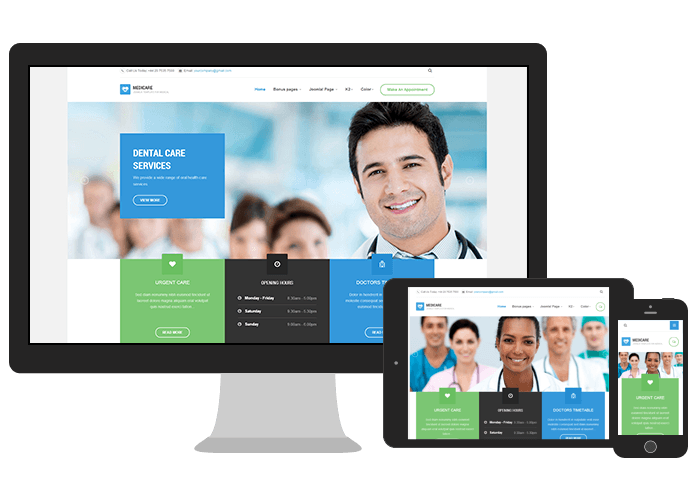In this image, three electronic devices—a computer monitor, a tablet, and a cell phone—are prominently displayed, each facing the viewer and turned on. All three screens showcase the same dental service website, featuring multiple doctors who are smiling warmly at the camera, creating an inviting and professional atmosphere. Amidst the friendly faces, additional website elements are visible, including sections for dental care services and urgent care options, along with glimpses of patients in the background, enhancing the context of a bustling, patient-focused environment. While the text on the website is blurry and difficult to read, the consistent imagery across all devices emphasizes a cohesive and welcoming presentation, underlining the accessibility and universal design of the dental service's digital presence.